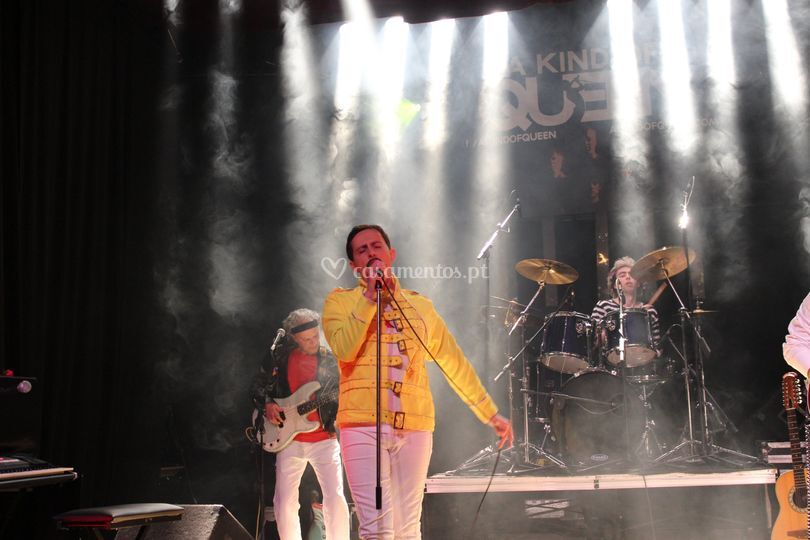This photograph captures a dramatic stage performance by what appears to be a tribute band imitating Queen. Central to the image is a performer strikingly similar to Freddie Mercury, donning his iconic yellow jacket with belt buckles and tight white pants, complete with his trademark mustache and brown hair. The singer passionately holds a microphone, embodying Mercury's presence. Directly beneath his chin, a watermark reads "cascamentos.pt" with a small heart next to it. 

The backdrop features vibrant, bright strobe lights with beams of light piercing through stage smoke, illuminating a banner partially obscured, which reads "A Kinder Queen." The drummer, positioned on a platform, wears a black and white striped shirt and has brown hair. To the left of the lead singer, an older guitarist with a white guitar is seen, wearing a red shirt, white pants, a black jacket, and a black bandana, standing in front of his microphone but not singing. On the far right, the arm and elbow of another musician are visible, alongside a guitar propped up against the stage structure. In the lower left corner, a keyboard and bench can be partially seen, indicating a comprehensive stage setup typical of rock concerts. The atmosphere, combined with the ensemble and flair of the performers, convincingly channels the energy and style of an authentic Queen performance.